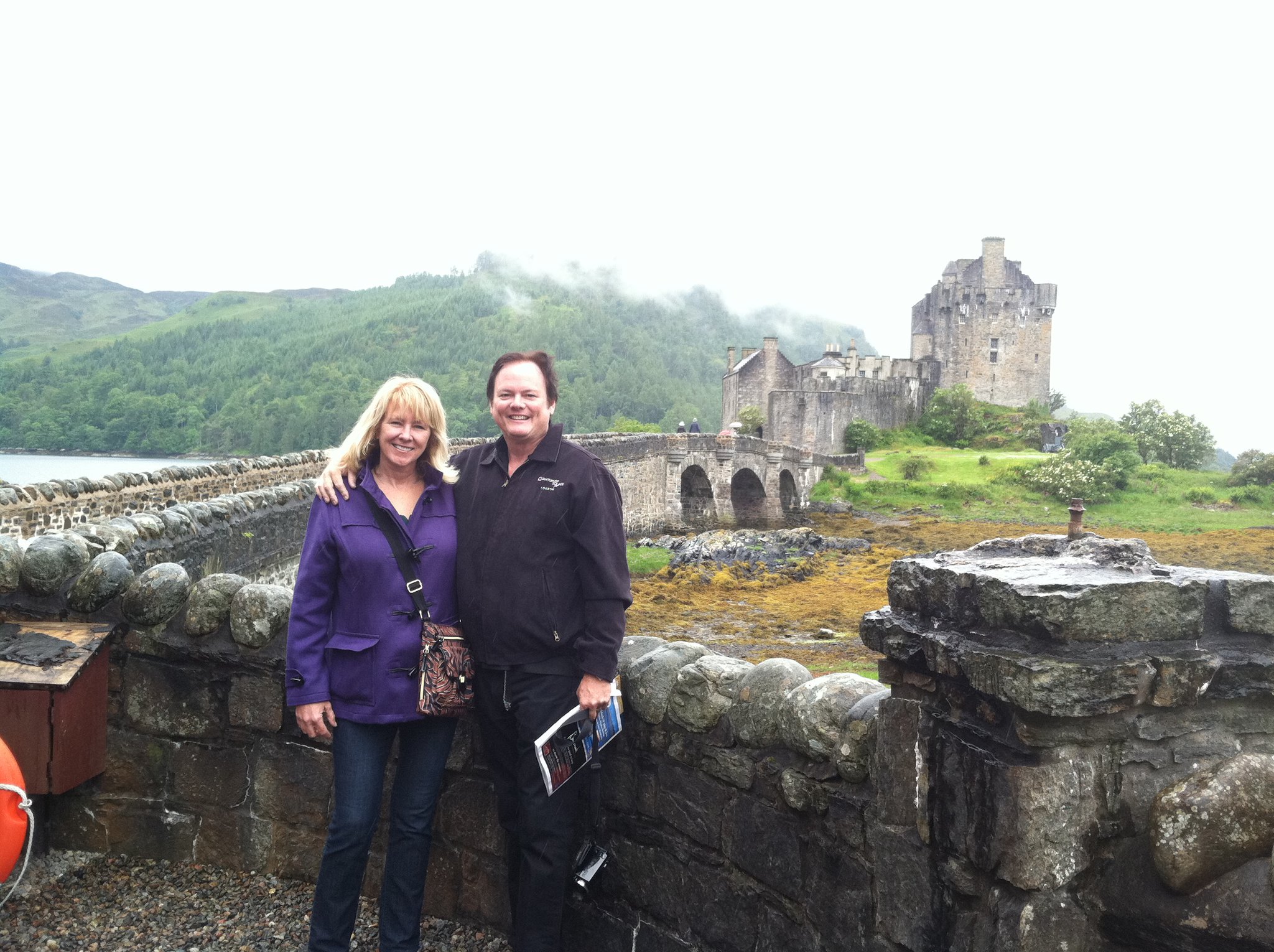A couple poses in front of a historic stone half-wall under a gray, overcast sky at a scenic European site. The man, likely in his 40s with short brown hair and a receding hairline, wears a zippered black jacket and black pants. He holds a pamphlet or tour guide and possibly a camera. His arm embraces a smiling woman with long blonde hair, dressed in a long-sleeve blue coat, carrying a purse, and wearing blue denim jeans. Behind them, a rustic bridge crafted from stone leads to an ancient, weathered castle with tan and gray hues, surrounded by lush greenery and forested hills. In the misty background, mountains rise up, adding to the picturesque landscape. On the far left, a small glimpse of water is visible, accompanied by a few people walking near the castle, enhancing the vibrant yet historic ambiance of the scene.